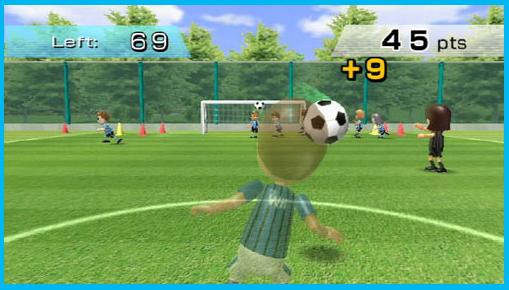In this detailed screenshot from a soccer video game, the scene showcases a vibrant, rectangular soccer field under a clear blue sky dotted with a few clouds. Towering green poles punctuate a giant fence that borders a line of trees encircling the pitch. At the forefront, a half-circle shapes the immediate foreground, featuring a translucent player with brown hair, wearing a black and green shirt and gray shorts, seen from behind and leaning slightly to the right.

To the right of this main player, a referee with short brown hair in black attire - composed of black socks, shoes, and clothing - gestures towards the other end of the field. Across the grass, seven soccer players, all in blue shirts with black shorts, are scattered, primarily concentrated near the opposite goal.

The field is also dotted with a white goal framed by orange cones. There's a soccer ball near this main goal, and another soccer ball visible in mid-air near the opposite goal. Notably, game information is overlaid at the edges of the screen: the upper left displays "left 69," indicating 69 seconds remaining, while the upper right shows the score with "45 points" and an additional "+9." Within the image, a light blue border frames the entire scene, enhancing the visual clarity of the gameplay.